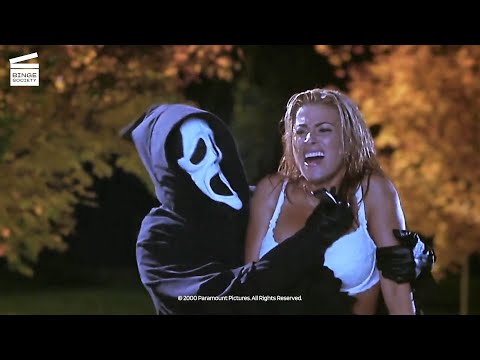This is an intense still shot from the iconic "Scream" movie series. The image captures a harrowing moment set at night in a dimly-lit backyard, evidenced by the dark sky and trees with orange-yellow leaves, suggesting it's fall. A menacing figure in a black hooded robe, donning the infamous white Scream mask with its gaping mouth, dominates the scene. The masked man, with black gloves, is violently stabbing a terrified blonde woman in the chest. She is barely clothed, wearing just a white bikini top, her face contorted in fear, and her mouth open in a scream. Her wet hair clings to her head, adding to the overall distress of the moment. In the lower part of the image, a text line reads "Paramount Pictures All Rights Reserved," grounding this chilling scene firmly within the realm of cinematic fiction.